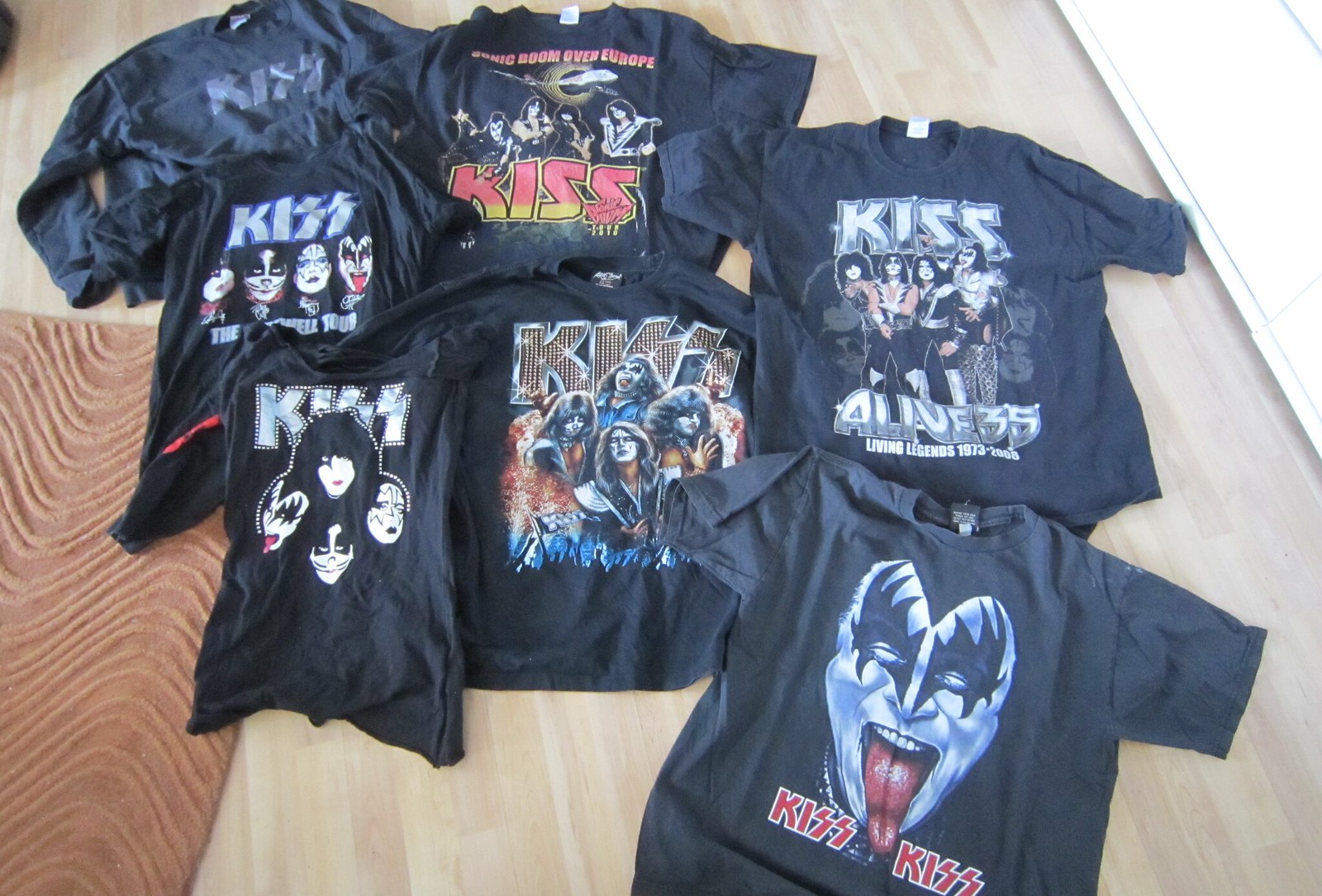This image showcases a collection of KISS band t-shirts, displayed on a light-colored wooden floor next to a light brown area rug with a swirly wave-like pattern. The shirts are predominantly black, with a variety of designs featuring band members in their signature makeup. One standout t-shirt depicts Gene Simmons with his tongue sticking out, while others highlight the entire band. The majority of the shirts have the word "KISS" emblazoned in white lettering with stylized "S's," though a few feature red, yellow, and sparkling gold variations. There is a mix of short-sleeve, sleeveless, and at least one long-sleeve shirt in dark gray. The arrangement appears slightly random, possibly indicating they're being prepared for sale, perhaps on eBay. The detailed graphics and iconic imagery make this a striking collection for any KISS fan.